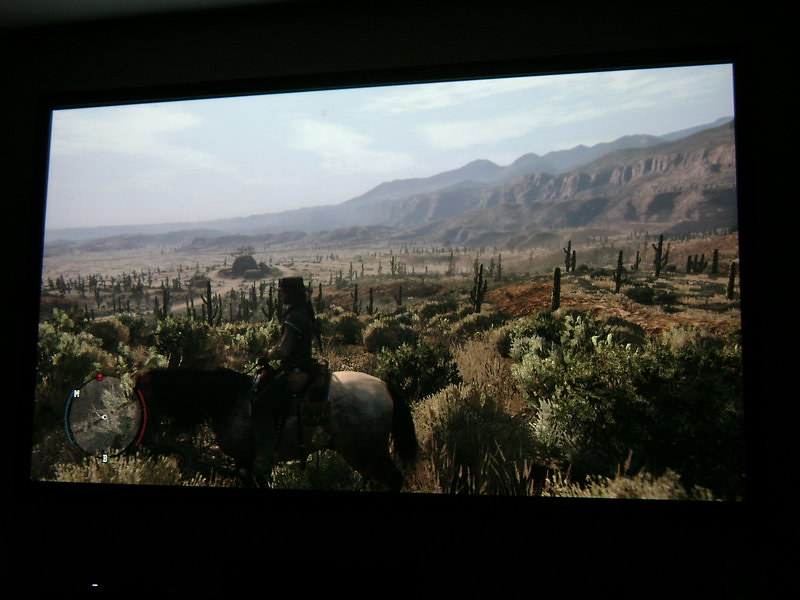The image captures what appears to be a high-resolution computer game displayed on a screen. Dominated by a deep black background, the lower left corner of the overall image features a small bright dot, suggesting a distant light source. The main screen showcases a vividly detailed Western landscape with a person on horseback navigating the terrain. The scene includes a rugged mountain range in the background, contrasted by cacti and shrubs in the foreground under a partially cloudy blue sky. A largely opaque compass at the bottom left corner of the screen indicates the character is heading west. The quality of the animation is exceptional, convincingly blending realism and artistic elements.